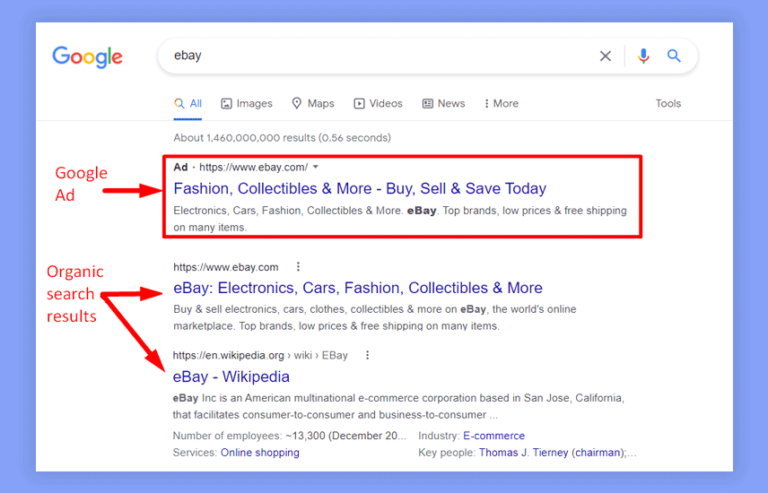This image depicts a screenshot of the Google search results page for the query "eBay." The background features a baby blue outer border and a white inner section. In the upper left corner, the Google logo is prominently displayed with its characteristic blue, red, yellow, and green lettering. The search box in the center contains the term "eBay," accompanied by an "X" for clearing the input, a microphone icon, and a magnifying glass search icon to the right.

Below the search box, the "All" tab is highlighted in blue, indicating that the user is viewing all search results. Additional tabs for "Images," "Maps," "Videos," "News," and "More" options, along with a "Tools" button on the far right, are also visible.

The search results summary indicates that approximately 1.46 billion results were found in 0.56 seconds. The top result is a Google ad for eBay, marked with "Ad" in red and highlighted by a red arrow within a box. The ad hyperlink reads "Fashion Collectibles and More - Buy, Sell, and Save Today," promoting eBay’s services and offerings such as electronics, cars, fashion, and collectibles with a note about top brands, low prices, and free shipping on many items.

Following the advertisement, there are organic search results. The first organic result is a hyperlink to the official eBay website, echoing similar promotional content. Below it is a link to the Wikipedia entry for eBay, which offers a brief description: "eBay Inc. is an American multinational e-commerce corporation based in San Jose, California, that facilitates consumer-to-consumer and business-to-consumer transactions." Additional details and hyperlinks are available further down the page.